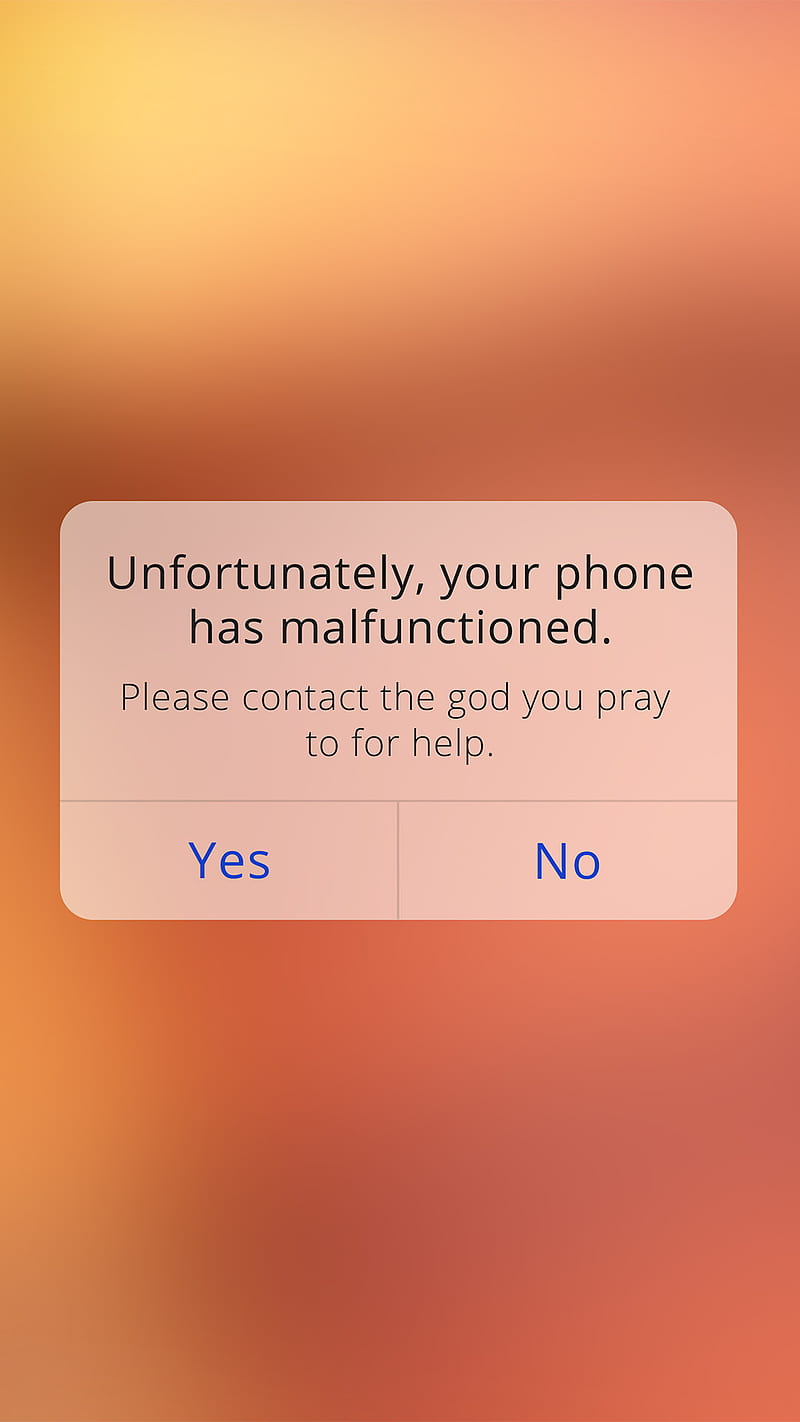The image showcases a vivid and abstract backdrop characterized by a gradient of colors. In the upper left corner, a soft yellow hue seamlessly transitions into a light orange and then into a salmon color in the upper right corner. As the colors progress downward, a band of darker pink is visible, gradually becoming lighter near the lower left corner where it fades back into yellow. Meanwhile, the lower right corner deepens into a darker pink shade.

Prominently displayed in the center of the image is a gray dialogue box. Inside the box, a bold black message reads, "Unfortunately, your phone has malfunctioned." Below this, in smaller, light gray text, is the phrase, "Please contact the God you pray to for help." At the bottom of the dialogue box, there are two blue response buttons: one on the left labeled "Yes" and the other on the right labeled "No."